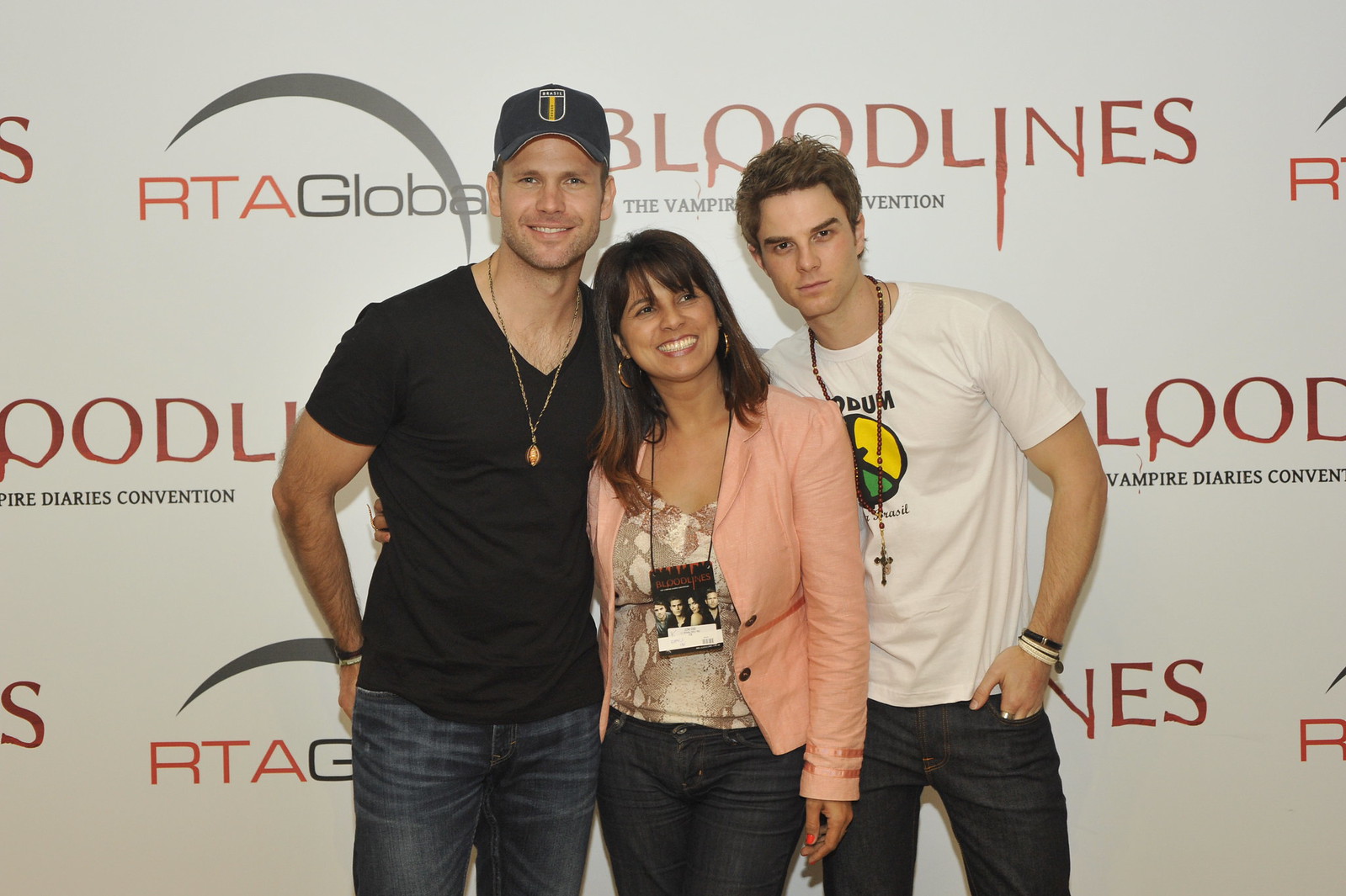In this image, three people are standing and smiling in front of a large white banner with dark brown letters that reads "RTA Global Bloodlines, The Vampire Diaries Convention." The banner features a crescent logo with RTA in orange and Global in gray. On the left is a man with a black V-neck short-sleeved shirt, a necklace with a charm, and dark blue jeans. He is wearing a blue hat with a logo and is smiling at the camera. In the center is a woman with shoulder-length brown hair, a big smile, and a beige and white shirt under a salmon-colored jacket. She has a lanyard around her neck, dark jeans, and looks enthusiastic. The man on the right is dressed in a white t-shirt with a large yellow and green symbol, a long necklace with a cross, bracelets on his arm (one black and two white), and dark jeans. He has short brown hair and is also smiling, looking happy to be there. The overall mood of the photo is joyful, with all three individuals excited to be at the event.